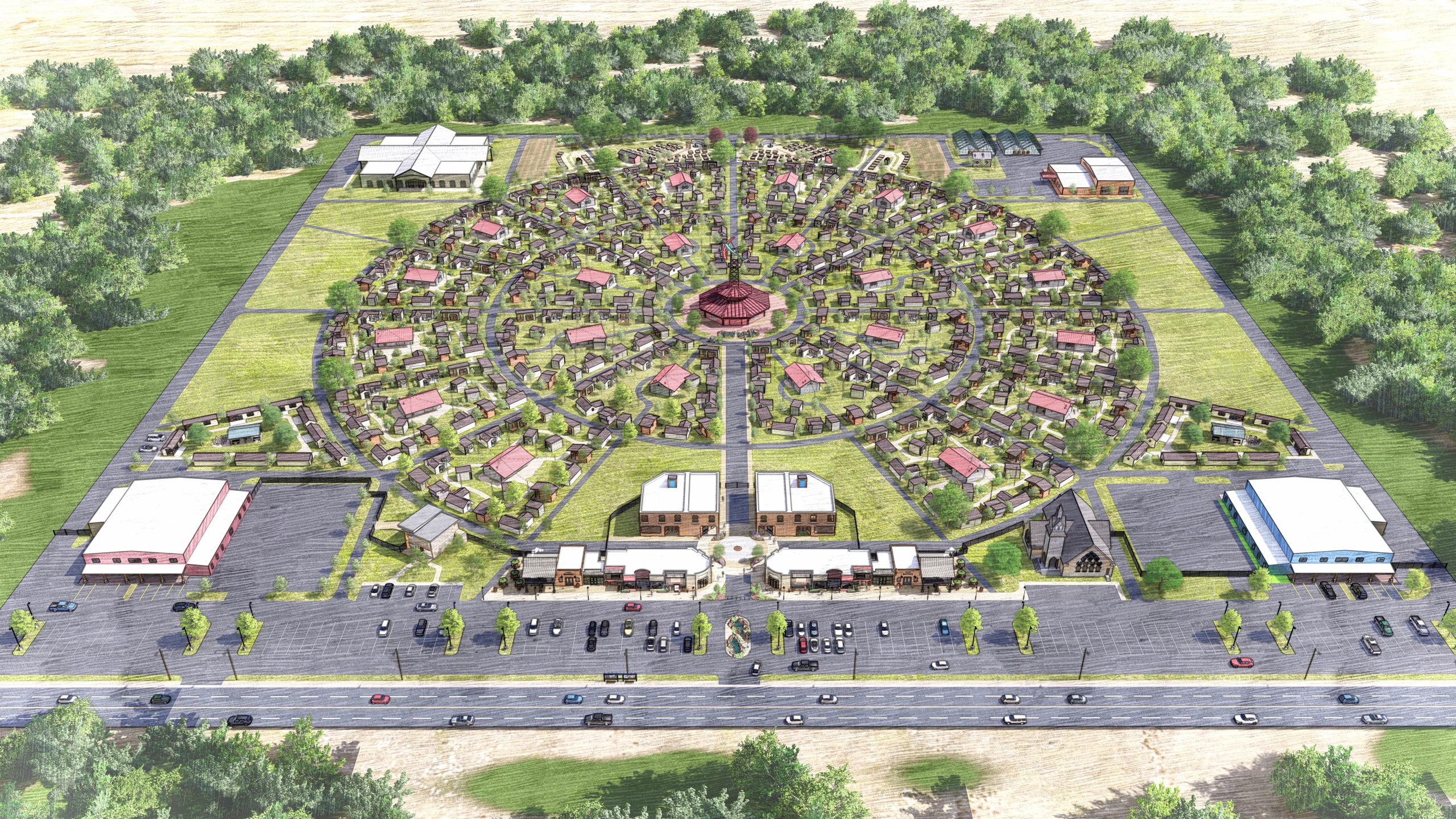The image is an outdoor illustration depicting what appears to be a meticulously planned small town or neighborhood centered around a prominent circular building, possibly a temple with a red roof. This central structure, which seems to be made of wood, is surrounded by various smaller buildings arranged in concentric circles, giving the area an almost spiral pattern. There are multiple rings of roadways or walkways radiating out from the center. The innermost ring hosts one large building with a red roof and several smaller white buildings with gray roofs. Beyond this, there are at least two more circular roadways, each encircled by more structures, including a mix of buildings with white and gray roofs. Encircling these rings is an outer square area with a mix of large and small buildings at each corner, some of which appear to serve as storage houses with white roofs, while others have gray roofs. The entire area is lush with greenery, including numerous trees, and features a parking lot with cars visible along the streets and nearby highway. The image is detailed and vividly uses greens for the grass and trees, emphasizing the organized, circular layout of this supposed temple complex surrounded by nature.